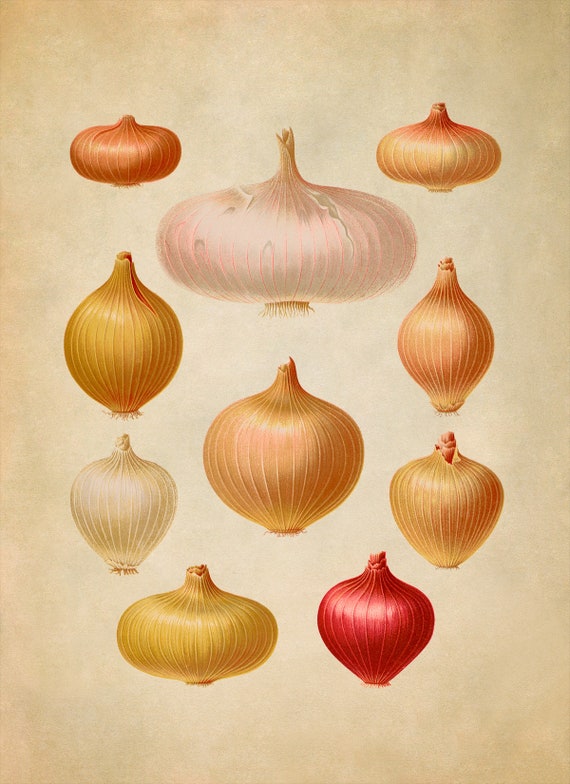This illustration, set against a uniform tan background that fades to white in the center, showcases various types of onions, each meticulously hand-drawn and colored. Predominantly clustered towards the middle of the image, a prominent white onion, streaked delicately with pink, is displayed slightly above a classic golden onion, creating a focal point. To the left of this central duo, there are four additional onions: a dark orange, a golden yellow with a top slit, a pure white, and another golden yellow. On the right side, four more onions are depicted: the top three exhibit hues of orange and yellow and vary in shape—from fat and short to thinner and bulbous—while the bottom one stands out as a rich, deep red onion. The harmonious arrangement and the subtle variations in size and color—from deep red to shades of gold and white—bring a captivating visual complexity to the artwork.